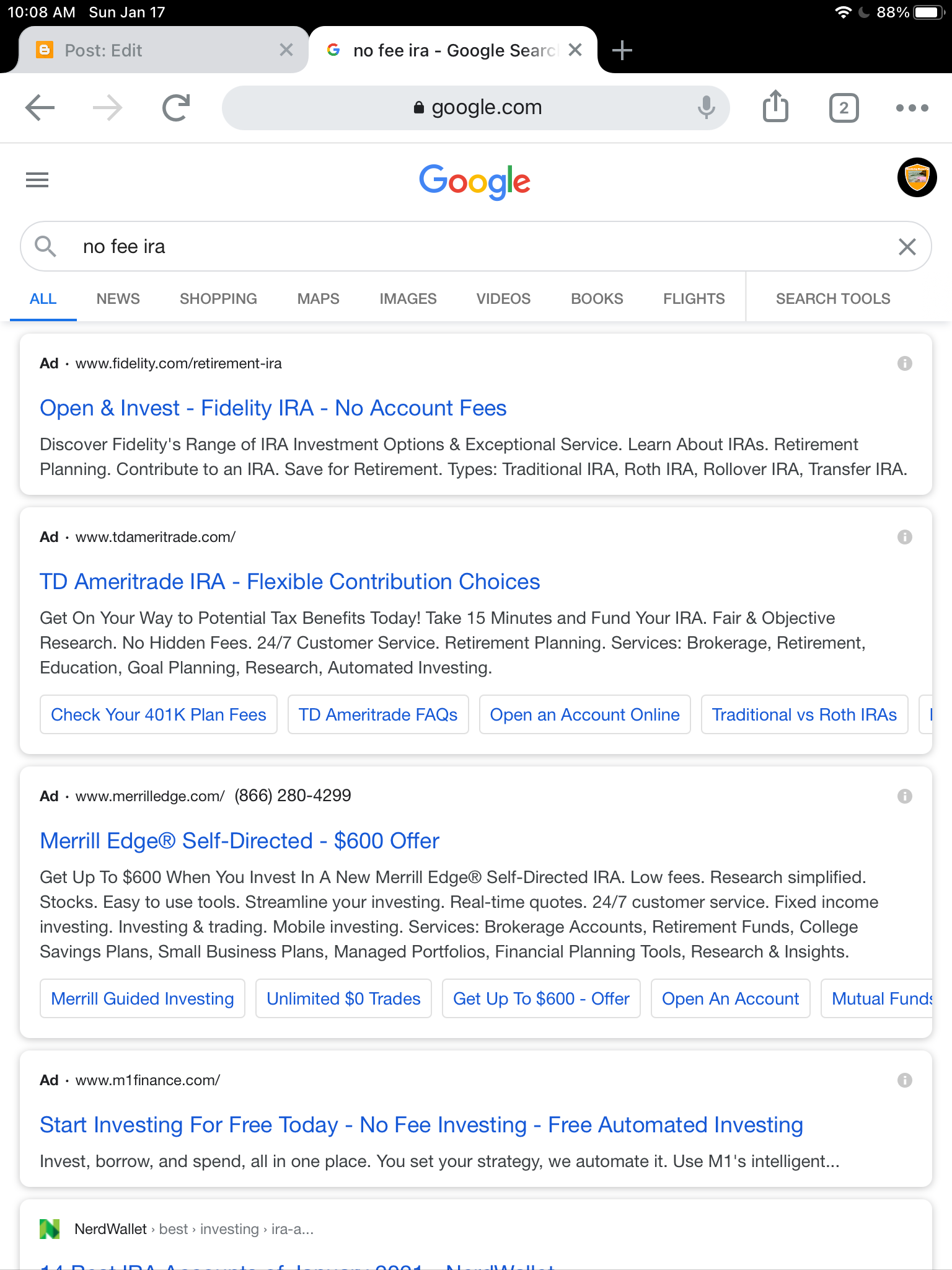This image is a detailed screenshot of Google's search results page taken at 10:08 AM on Sunday, January 17th. The top of the screen features a black bar where the device's status icons are displayed on the right side, showing a Wi-Fi connection icon and a battery level at 88%. To the left, in white, the date and time are clearly marked.

The browser shows two open tabs: one on the left labeled "post edit," which is greyed out, and the active tab on the right is Google's search page. The search query, "No fee IRA," is entered into the Google search bar, which also includes navigation arrows and a reload icon. 

Below the search bar is a typical Google layout with the company's logo on the left and a small round profile icon with a face on the right, next to a "hamburger menu" symbol. The search results are contextualized under various tabs: "All," "News," "Shopping," "Maps," "Images," "Videos," "Booking," "Flights," and "Search tools," with "All" visibly selected and highlighted in blue.

The search results begin with the following entries:

1. **Fidelity Investments:** The blue link reads, "Open, invest, Fidelity, IRA, no account fees." The snippet highlights Fidelity's range of IRA investment options, exceptional service, and details about different types of IRAs, including traditional, Roth, rollover, and transfer IRAs.

2. **TD Ameritrade IRA:** This link reads, "TD Ameritrade IRA, flexible contribution choices." It promotes potential tax benefits, quick account setup, no hidden fees, continuous customer service, retirement planning services, brokerage, education, goal planning, and automated investing. Sub-links provide more resources such as "Check your 401k plan fees," "TD Ameritrade FAQs," "Open an account online," and "Traditional vs. Roth IRAs."

3. **Merrill Edge Self-Directed:** Advertising a "$600 offer," this result presents additional text and clickable boxes for further exploration.

4. **Start Investing for Free Today:** The final visible entry suggests no-fee investing and free automated investing options.

The screen is slightly cut off at the bottom, leaving part of the search results obscured. The URLs of these links are not fully visible due to their small size in the screenshot.